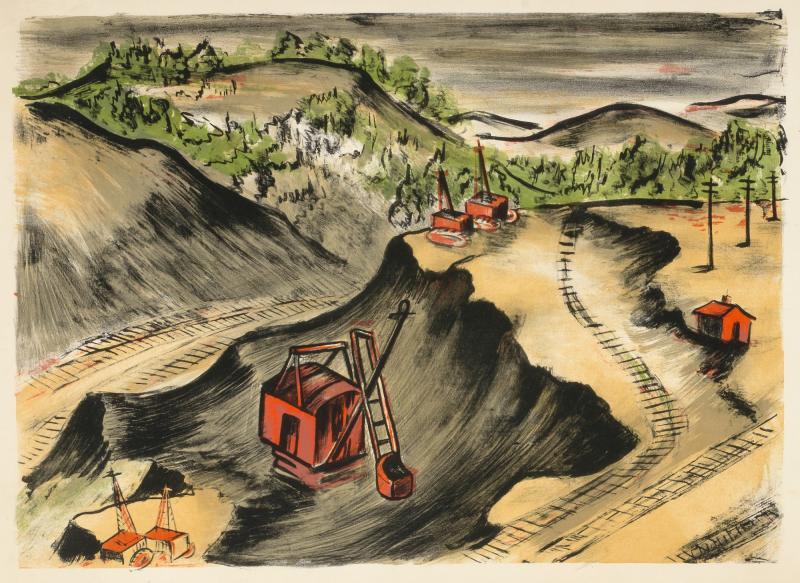This detailed illustration, reminiscent of a vintage child's picture book with a somewhat childlike and old-fashioned style, depicts a gloomy construction site set against a backdrop of mountains and trees under gray, charcoal-lined skies. The scene is filled with shades of black, gray, and beige, punctuated by the notable presence of red, peachy, and pinky-orange hues. Prominently featured is a red piece of construction equipment with a digging bucket, and two additional, less distinguishable pieces of red machinery. The foreground showcases a pale gold patch of excavated land, marked by vehicle tracks and a significant dug-out hole. Train tracks curl on both sides of the image, enhancing the industrious atmosphere. A small red house and three telephone poles devoid of wires add to the rustic charm of the setting. The overall composition suggests a busy yet melancholic early morning at this sprawling excavation site.